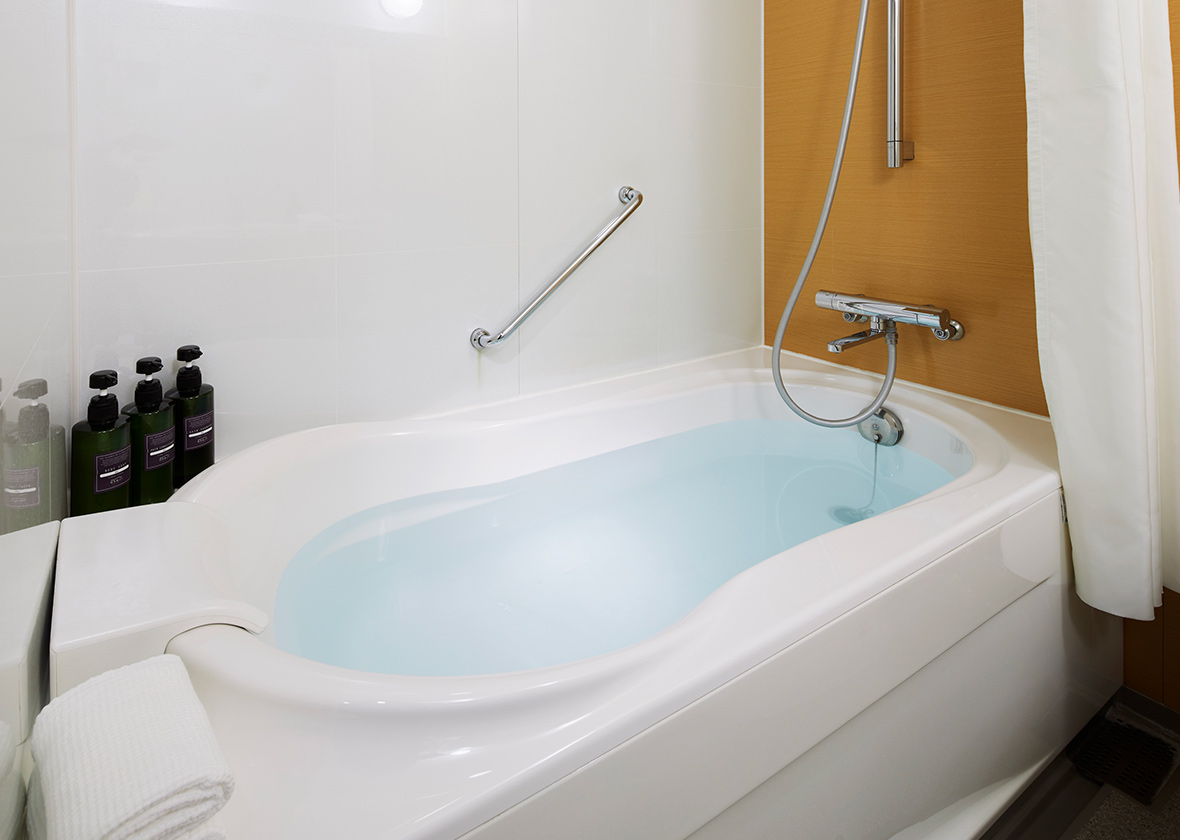The image depicts an inviting, modern bathroom that could be part of a hotel or a private home. At the center is a large, white porcelain bathtub filled with light blue water. The tub features modern chrome fixtures including a faucet and a plug. For accessibility, there are chrome grab bars on the side wall, which is tiled white. Adjacent to the tub is a darker brown wooden wall adding a touch of warmth to the setting. 

On the right side, there is a set of three black pump bottles potentially containing shampoo, body wash, and conditioner. Below them, a neatly folded white towel rests at the foot of the tub. To the far right, a white shower curtain hangs down. The sleek design and these thoughtful elements make the space feel luxurious and ready for a relaxing bath.